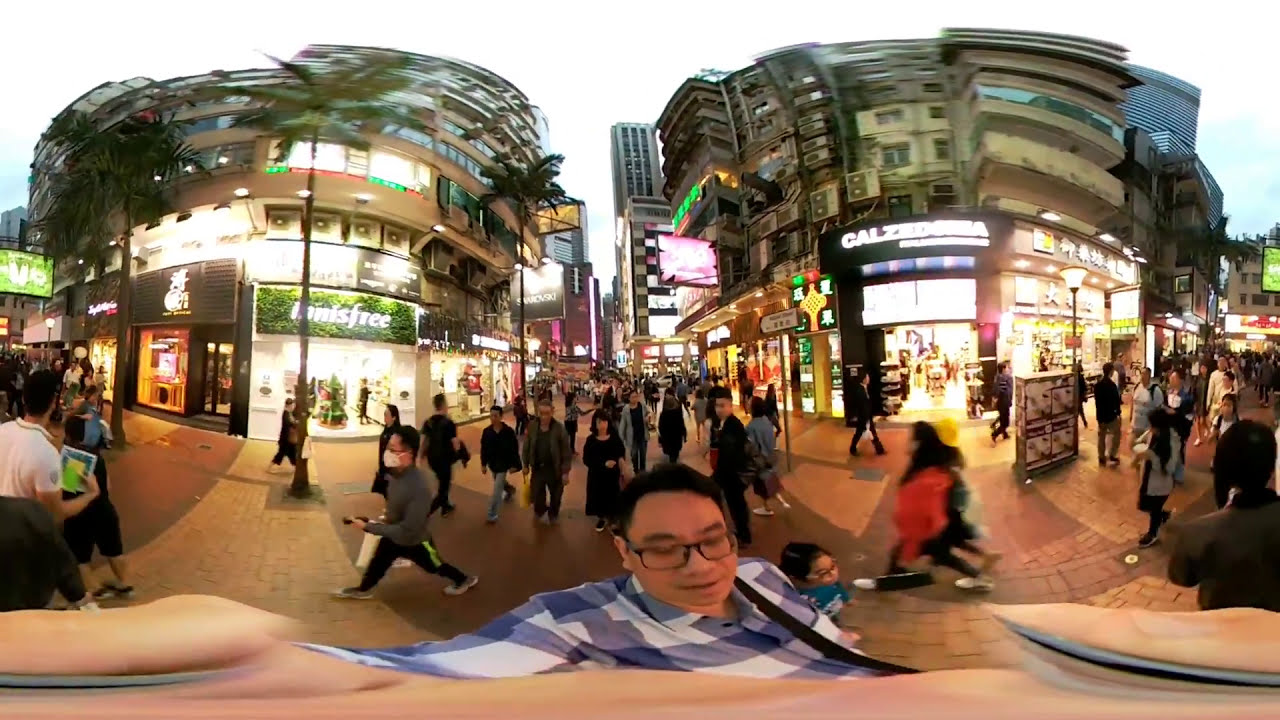The photo captures a bustling city scene, likely in an Asian metropolis. It is a selfie of a man in glasses, sporting a blue and white striped shirt. He is seated at what appears to be an outdoor mall, with brick walkways and numerous people walking around him. The atmosphere is vibrant and lively, illuminated by bright lights from multiple tiered stores. 

To the center left, the man takes the photo, while various tourists and locals meander along the walkways, some wearing light jackets, suggesting mild, comfortable weather approaching evening. Distinct signs in Asian languages and store advertisements are prominent, indicating a non-English-speaking country. 

In the background, towering skyscrapers and city buildings blend into a busy streetscape filled with uncountable pedestrians. Notably, to the right, a store shines brightly, with possible names starting with "C" or "A" and displaying Asian characters. Another similarly large and tiered store to the left, possibly named "tennis-free," features open doors and visible interior decor, contributing to the lively, cosmopolitan ambiance.